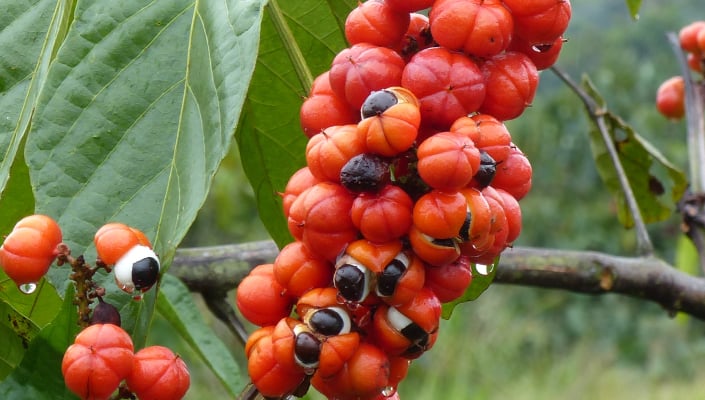This close-up outdoor photograph features a cluster of red guarana berries at the center, prominently displayed amidst a backdrop of blurred grass and trees. The berries, which resemble small pumpkins or cherry tomatoes due to their distinct ridges and vibrant red color, are growing from a branch surrounded by large, broad green leaves. Several of the berries have burst open, revealing their unique interior: a striking white shell encasing a dark, black seed that resembles an eye. While most berries remain intact, a few split ones, including a prominently extruding one on the far left, are clearly visible. The background is filled with additional and partially visible berry clusters, providing a lush, tropical context to the image.